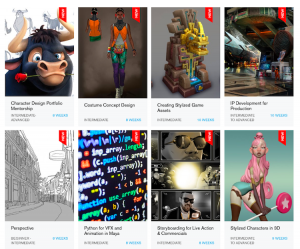This rectangular collage consists of eight distinct images arranged in two rows of four. Here’s a detailed breakdown:

1. **Top Left Image:** A striking illustration of a bull with a rose in its mouth. The bull has black fur, white horns, and intense white eyes. There appears to be some text underneath the bull, but it's too small to decipher.

2. **Top Second Image:** A graceful female figurine that seems to be a video game character. She is standing confidently, and behind her, there is an additional outfit displayed.

3. **Top Third Image:** A mystical scene showcasing what looks like an Aztec temple. Water cascades down from the structure, crowned by a prominent head sculpture at the top.

4. **Top Right Image:** An enigmatic structure that resembles a building. The specific details are unclear, indicating it could be an abstract or artistic representation.

5. **Bottom Left Image:** A nostalgic black-and-white photograph capturing an old city street, evoking a vintage charm.

6. **Bottom Second Image:** A screen filled with lines of programming code, suggesting themes of technology and computing.

7. **Bottom Third Image:** A vibrant comic book-style illustration portraying a character with glasses, exuding energy and dynamic action.

8. **Bottom Right Image:** A striking anime portrayal of a female character with pink hair, who gazes directly at the viewer with an engaging and expressive look.

Each image contributes a unique visual element, ranging from art and architecture to technology and animation, forming a diverse and rich collage.